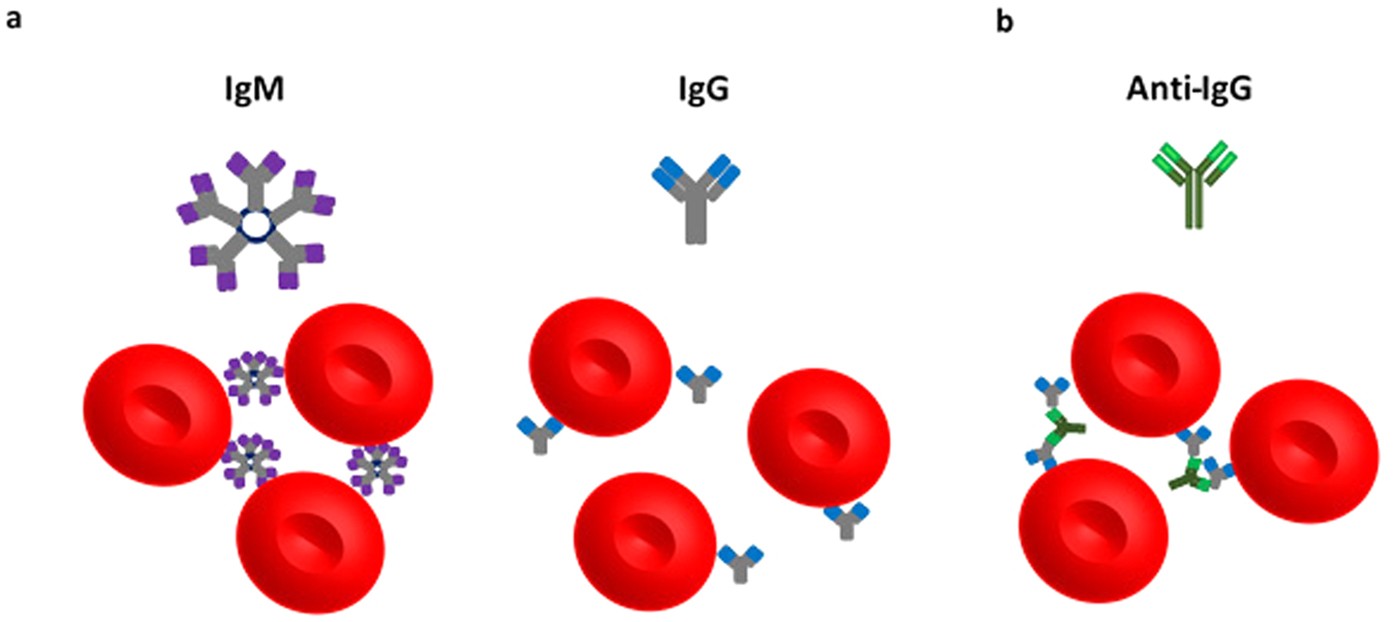This image is a detailed diagram illustrating the different forms of immunoglobulins (IgM, IgG) and anti-IgG antibodies and their interactions with red blood cells. On the left, labeled with the letter 'A', is the IgM molecule, depicted as a pentameric (five-pointed star) structure, with each point branching out into a V-shaped formation with two purple tips. This IgM structure is shown binding to three red blood cells below it. In the middle section, labeled with 'B', is the IgG molecule, characterized by its Y-shaped structure with blue tips. The IgG molecules, four in total, are illustrated attaching to red blood cells beneath them. On the right, the anti-IgG, also a Y-shaped molecule but entirely green with lighter green tips, is depicted. The anti-IgG antibodies are shown binding to the IgG molecules attached to the red blood cells, demonstrating the interaction between them. Throughout the image, the red blood cells are consistently represented as red circles with a central indentation, reflecting their biconcave shape.